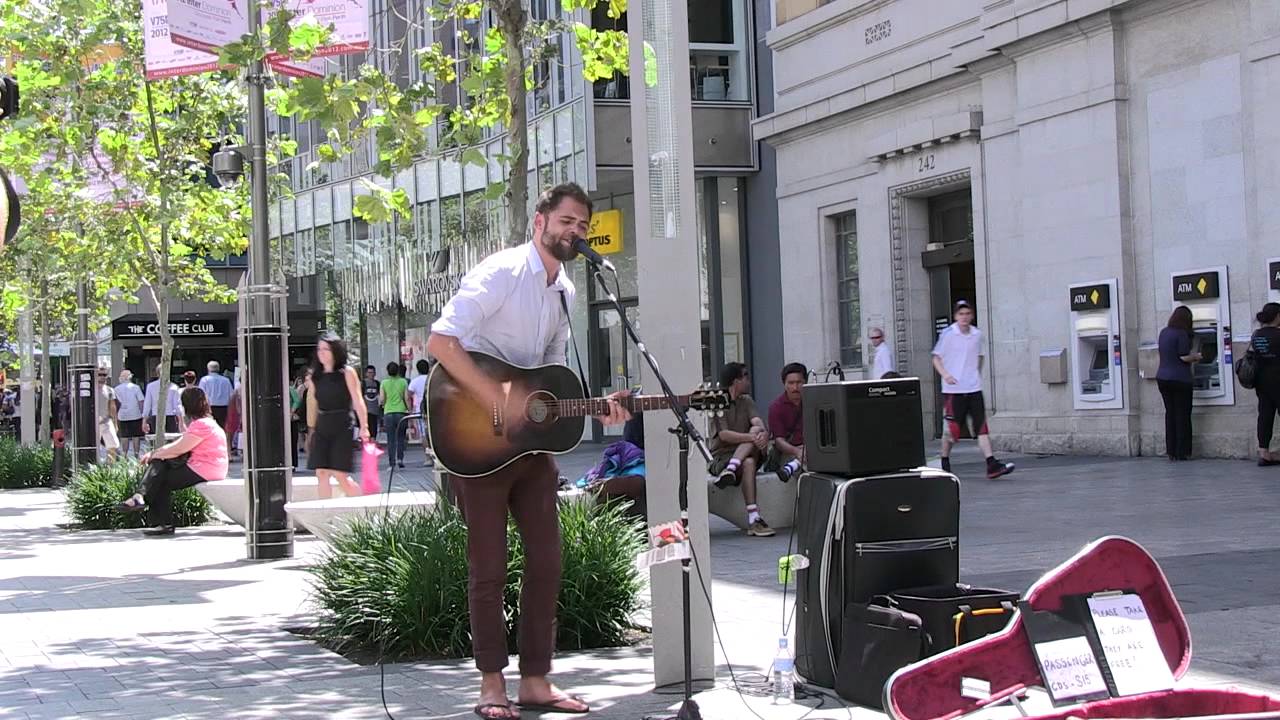The photo depicts a street musician, a tall man with short brown hair, a goatee, and a beard, playing an acoustic guitar and singing into a microphone. He is wearing a white button-up, collared shirt with brown trousers and sandals. The guitarist has his red-lined guitar case open for donations and is accompanied by a setup of amplifiers. The scene unfolds in a bustling outdoor area adorned with green shrubs and surrounded by a variety of people. To his left, a cluster of individuals is seen walking toward "The Coffee Club," a gray concrete building. To his right, along another concrete structure with multiple windows, people are using ATM machines. Additional details include a man in shorts with a white shirt observing the performance and two women, one in a black dress and another in blue jeans with a green polo shirt, also present in the vicinity. The atmosphere is lively with an evident blend of art and urban daily life, all under the daylight.